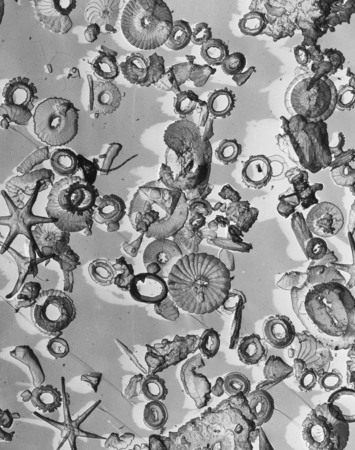This image portrays a grayscale beach landscape, densely populated with various seashells, starfish, and circular objects scattered randomly across a gray background. The starfish, notable for their six arms radiating from the center, appear prominently throughout the scene. Numerous circular shapes, some resembling seashells with intricate, circular indentation lines, and others appearing as dark rings or donut-like forms, are scattered around. The arrangement, which seems haphazard and unorganized, gives the impression of a detailed, almost microscopic view. Some of the objects have a white outline, adding to their visibility and definition against the varying shades of gray. The mix of detailed textures and shading, along with the varied patterns and shapes, creates an intriguing and complex visual experience.